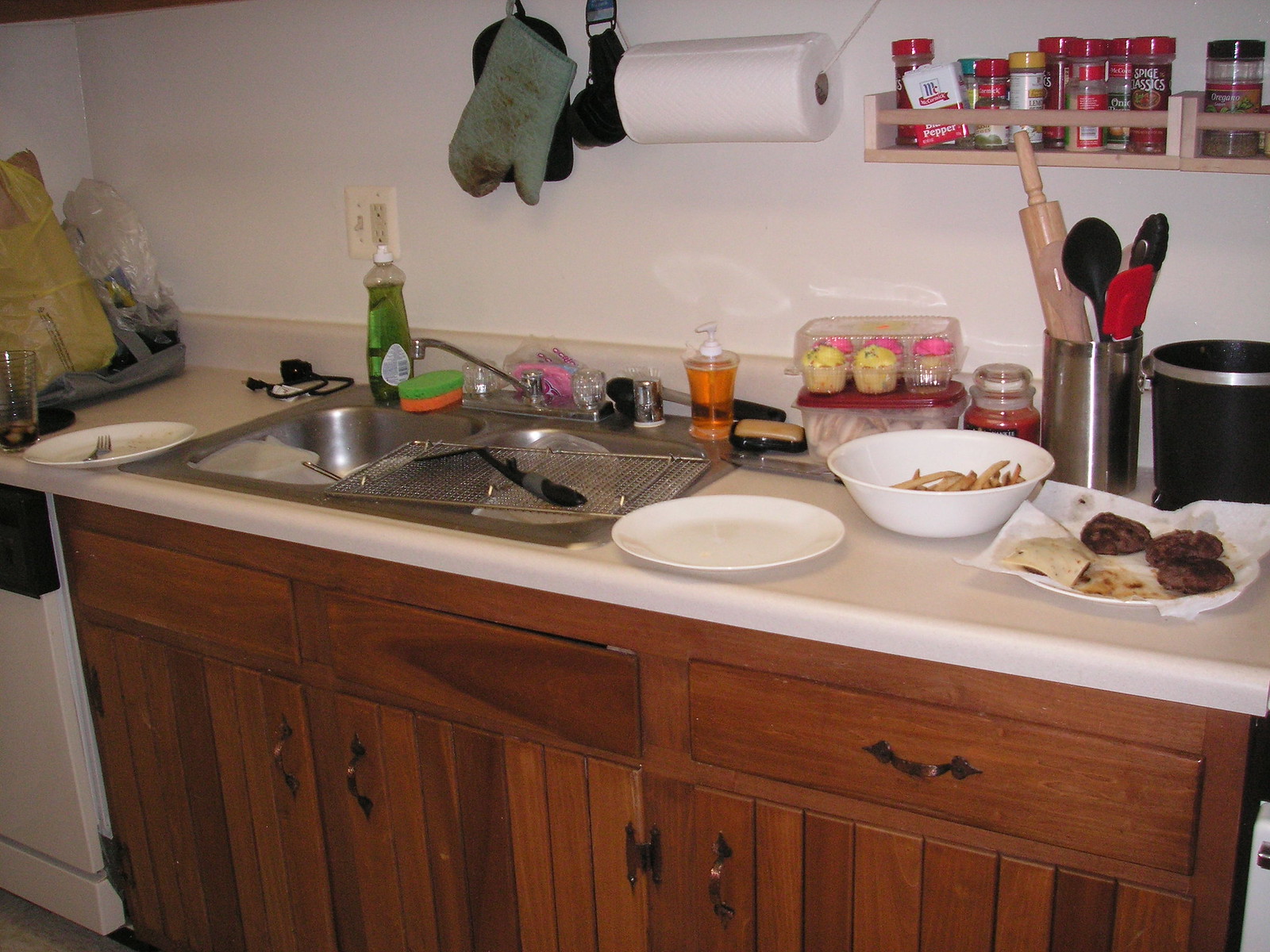This image captures a messy kitchen sink scene. The sink, constructed of silver metal, is cluttered with dishes and kitchen utensils. In the forefront, there are three white plates stacked alongside a white bowl. Positioned within the bowl are what appear to be French fries. Directly on the sink sits a metallic strainer holding a spatula. 

To the right of the bowl, three burgers rest on paper towels, likely placed there to absorb excess oil. In the background, a transparent plastic pack of muffins is visible. Originally holding six muffins, the pack now contains five. The front two muffins are yellow and could be banana-flavored, while the three at the back are adorned with pink icing.